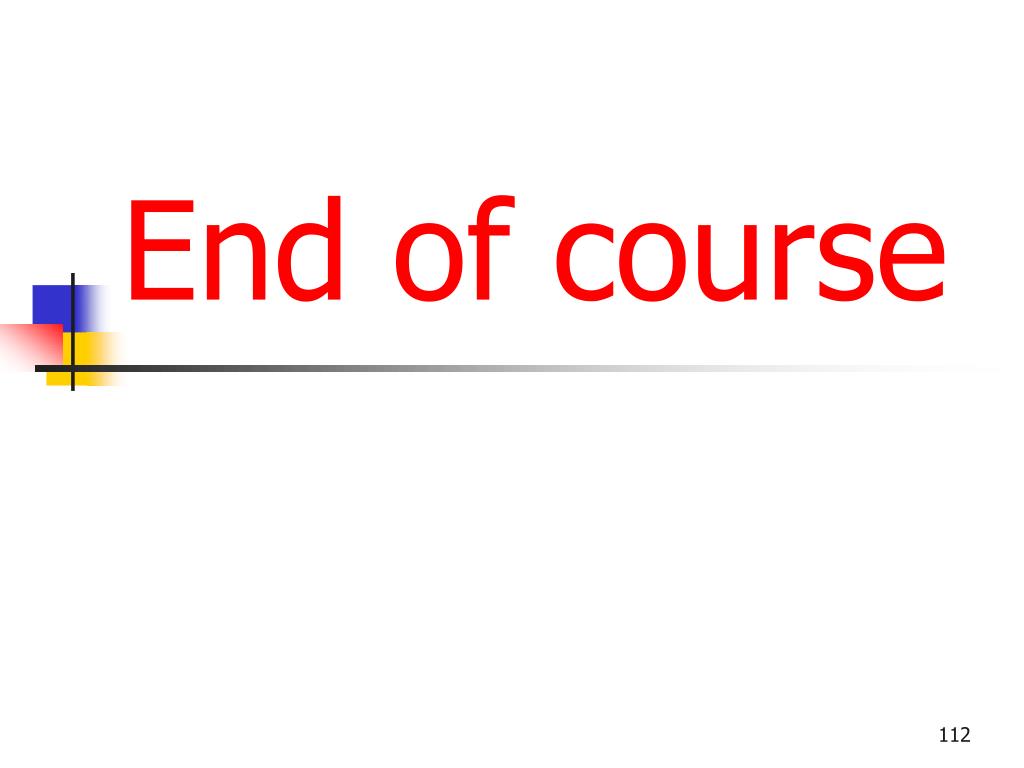The image features a white background with prominently displayed red text in the center that reads "END OF COURSE," written in capitalized letters and in a Helvetica font. The text is underlined by a continuous black line. In the bottom right corner, the number "112" is printed in small, black text, which could indicate a slide number. The lower left corner showcases a logo consisting of three overlapping rectangles in red, yellow, and blue with intersecting black lines running vertically and horizontally through them. The design elements suggest that this could be the final slide of a presentation or a scanned page from an educational textbook or website.